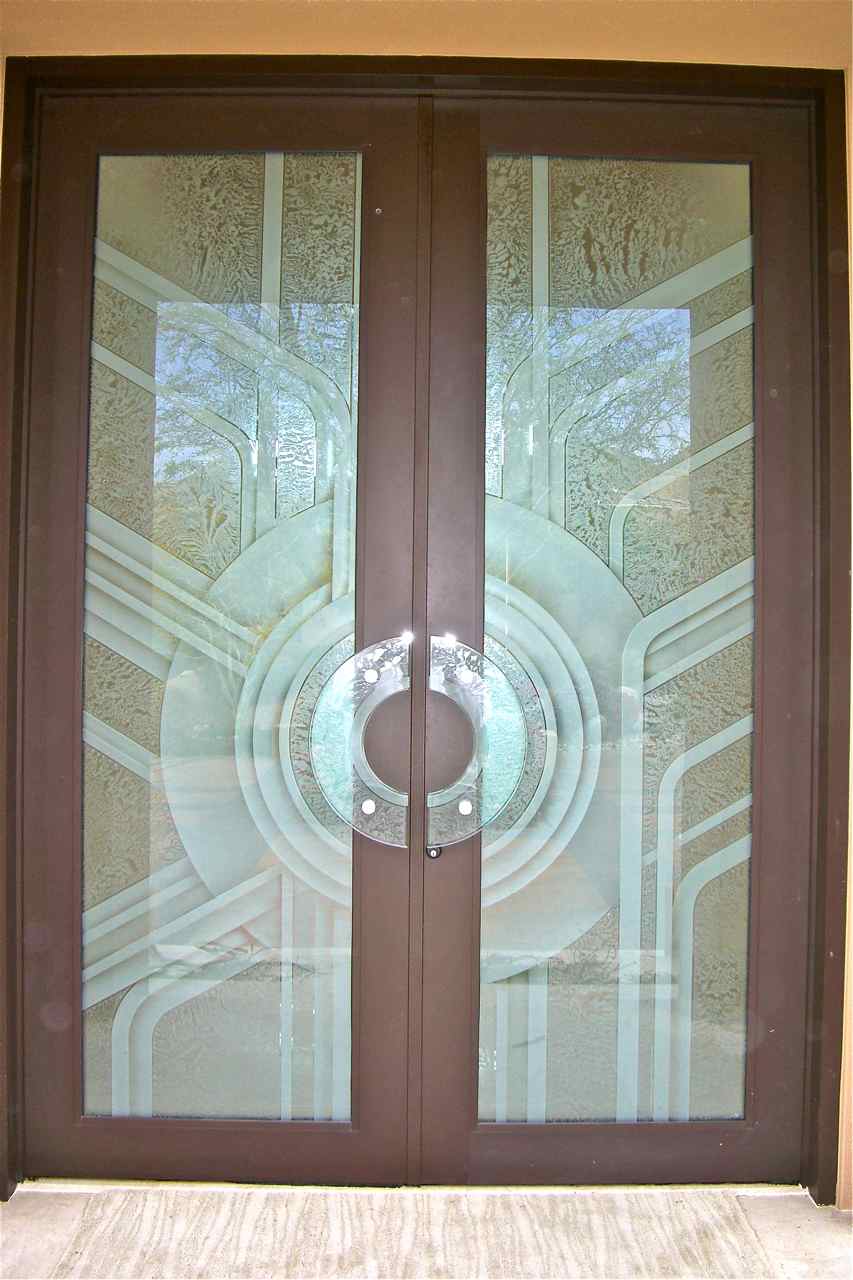This photograph captures a double-glass door framed by dark wood. Each panel of the door is encased in a thick wooden frame stained a rich, dark reddish chocolate brown. The building surrounding the door is visible at the top of the image, showcasing a dark sandy color. Below, the walkway leading up to the doors consists of gray bricks or paving stones. The glass panels within the doors feature intricate, geometric designs with a mechanical aesthetic, highlighted by a large central circle. This central motif is complemented by two half-circle glass door handles mounted directly onto the wood. Reflecting in the glass, one can see a vivid blue sky and some trees positioned behind the photographer, adding a touch of natural beauty to this architectural detail.